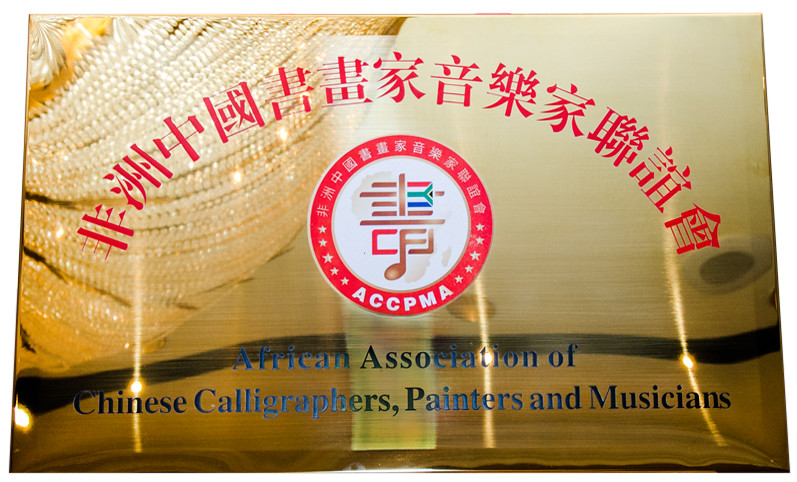The image features a prominent logo positioned directly in the center, set against a backdrop that resembles either a company sign or a glass window in a building. The logo consists of a red, semicircular design that includes Chinese text and the acronym ACCPMA. Above and around the logo are additional pieces of text in various Asian languages, which enhance its intricate design. The acronym stands for the African Association of Chinese Calligraphers, Painters, and Musicians, which is spelled out at the bottom of the logo in blue text. The entire scene is awash with vibrant colors including yellow, tan, red, blue, green, purple, and brown. To the top left of the image, there is a piece of stitched fabric, adding a textured element to the otherwise sleek and professional design.